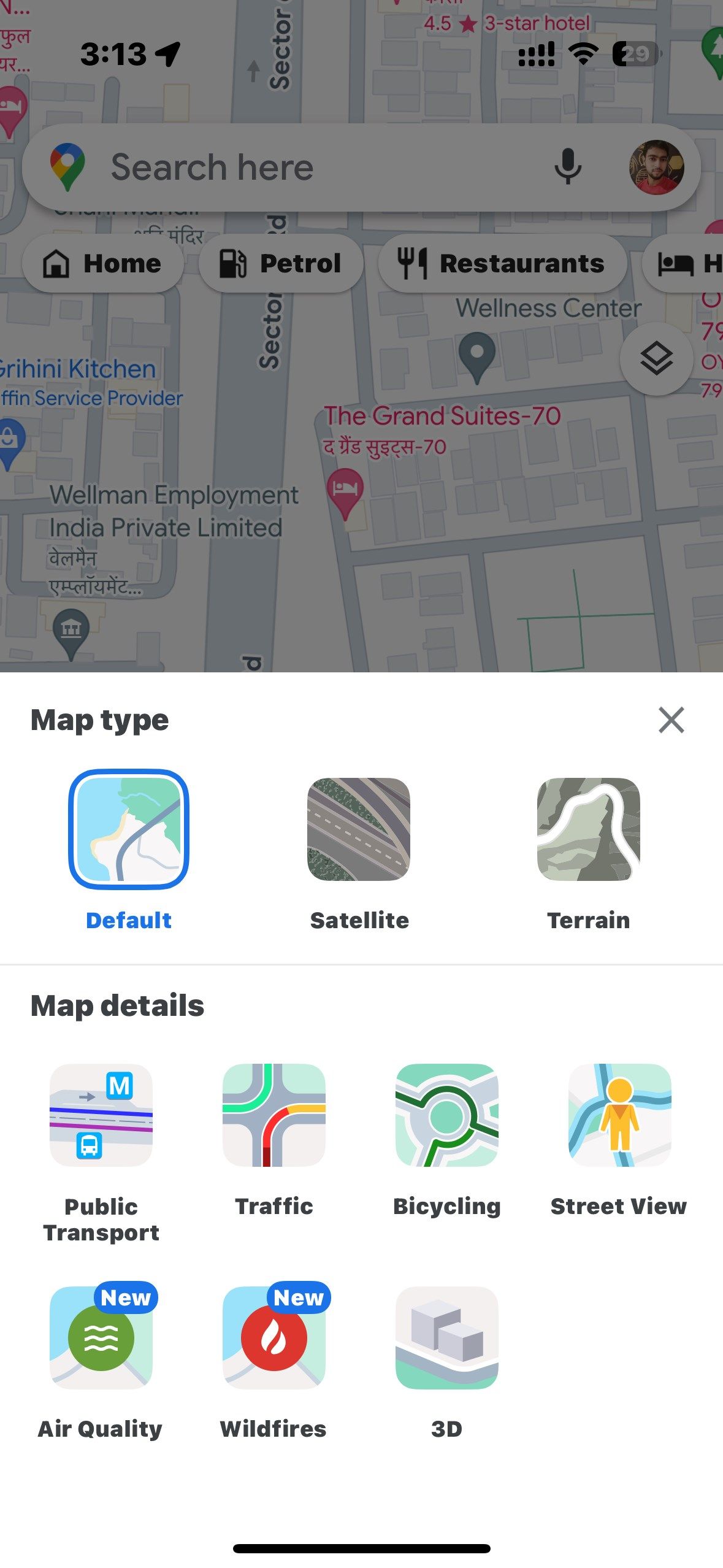This image is a screenshot from what appears to be an off-brand map application, possibly similar to Google Maps. At the top of the screen, there is a square displaying a section of the map with a gray filter applied. The top-left corner indicates the time as 3:13 and shows that location sharing is active. The user has full Wi-Fi and mobile signal, and their battery level is at 29%. Just below this, a roadmap is visible, highlighting Sector Avenue. A search field with a microphone icon is present alongside the user's profile picture, which features a 20-something-year-old Middle Eastern man.

Further down, there are clickable menu options labeled "Home," "Petrol," "Restaurants," and "Hotels." The map depicted seems to be of an area in India, as evidenced by the display of "Wellman Employment India Private Limited" and other annotations written both in Hindi and in English. At the bottom of the screenshot is a white rectangle offering different map view options: Default, Satellite, and Terrain. The Default view is currently selected.